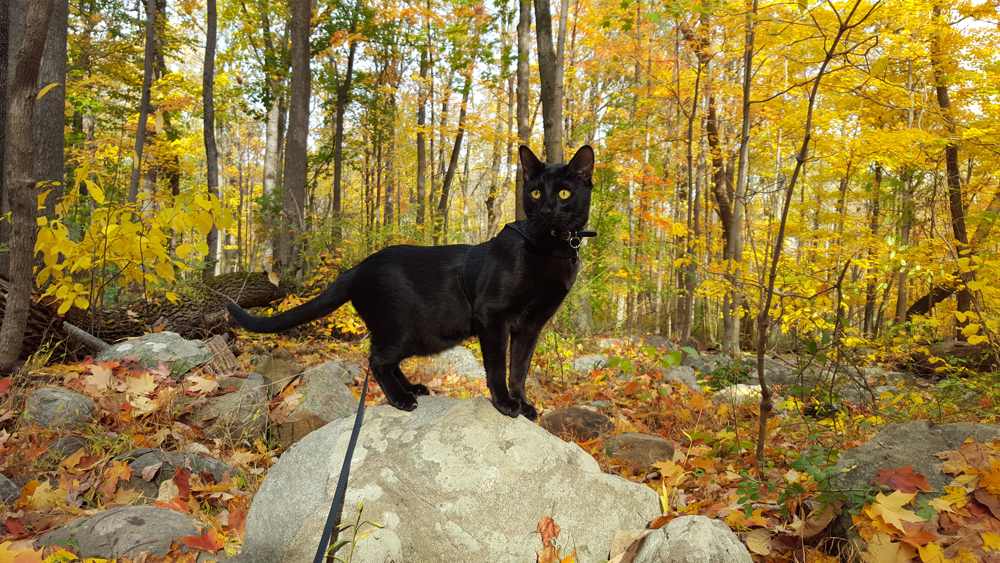In this horizontally aligned rectangular image, an impeccably groomed black cat stands in profile on top of a large, light gray rounded boulder. The cat, wearing a collar, is positioned slightly off-center towards the left and looks off into the distance, with its head turned forward slightly to the left. Its light yellow-green eyes and erect ears give it an alert expression against the backdrop of a serene autumnal scene. The area is a wooded setting with many tall, narrow tree trunks adorned with yellow, orange, and some remaining green foliage. Scattered across the ground are numerous fallen autumn leaves in red, orange, and yellow hues, covering the surrounding rocks and boulders. Some weeds poke through these rocks and leaves, adding to the natural, unkempt look of the forest floor. Patches of clear sky peek through the tree branches, indicating a bright, clear day. The cat’s slender, solid black frame and long tail contrast strikingly with the white and brown tones of the boulder it stands on, creating a captivating focal point amidst the scenic autumnal environment.